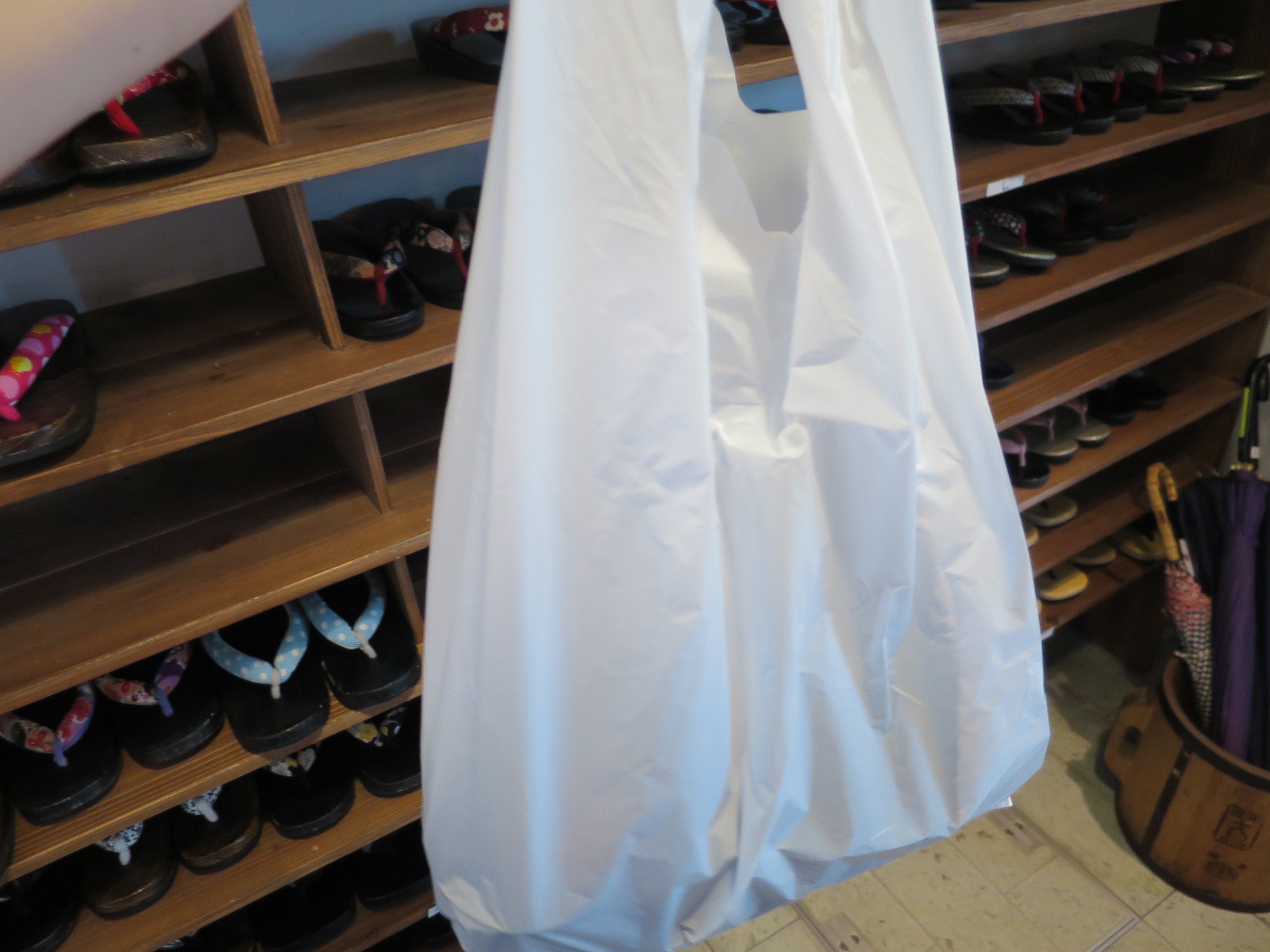The image depicts a neatly organized shoe store, predominantly showcasing beach-style flip-flop sandals. The sandals are displayed on a wooden shelving unit that extends ten rows high, with various slots to house the footwear. While the designs feature a range of colors including blue, pink, black, red, and green, they all share a common floral pattern. In the front center of the image, someone is holding a white plastic bag with their left hand, its contents weighing it down. To the right, there is a distinctive umbrella holder shaped like a giant wooden mug, containing several umbrellas and canes. The scene is set atop a floor with a wood grain finish, adding a rustic touch to the vibrant display.